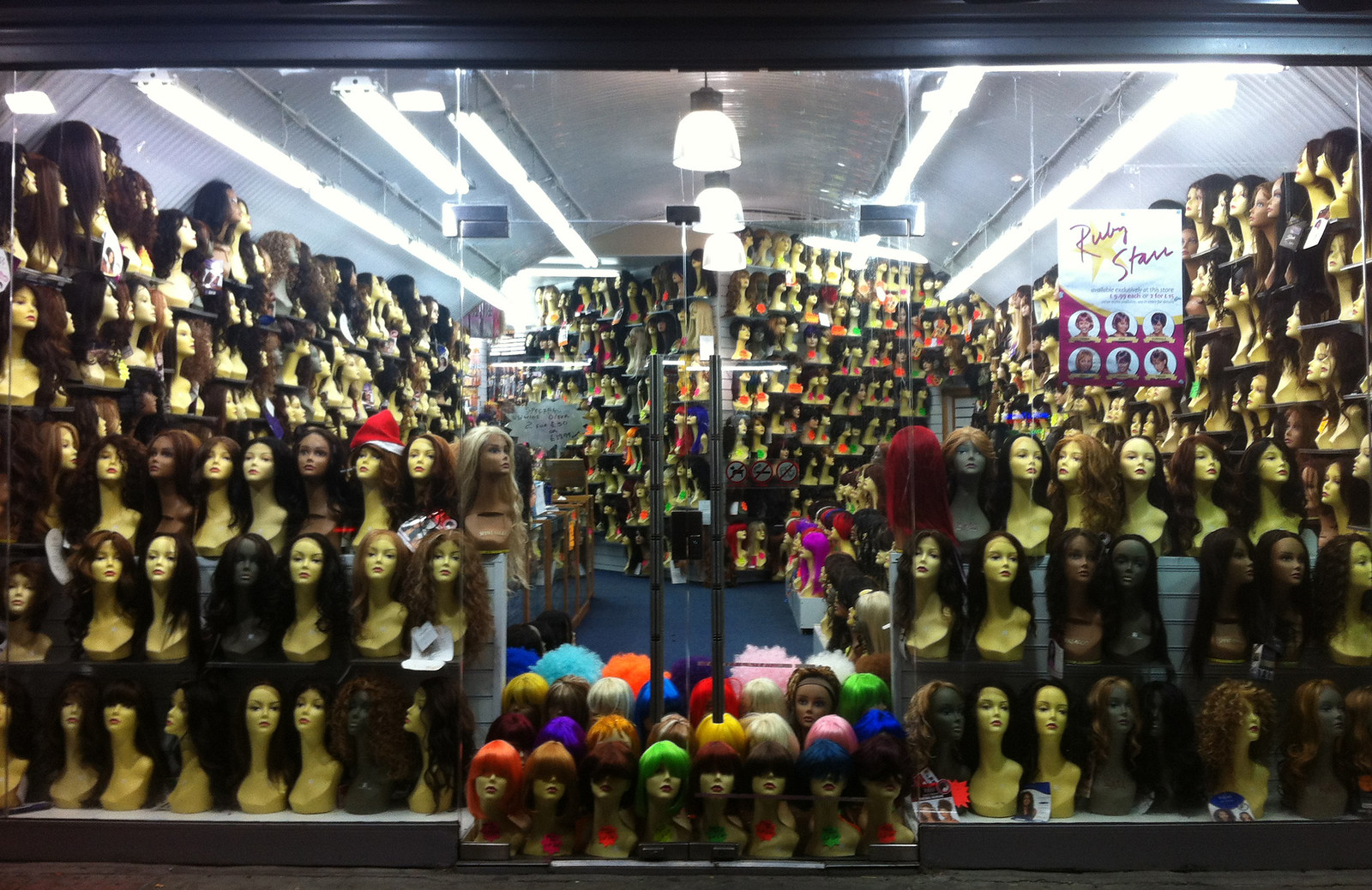The image is a horizontally oriented, nighttime photograph of a brightly illuminated wig shop, captured from outside through the large plate glass window of the storefront. Inside, the store is long and narrow, with rows of floor-to-ceiling shelves absolutely packed with mannequin heads displaying an overwhelming variety of wigs. The wigs come in all colors and styles, showcasing a spectrum from natural brunette and blonde to vibrant neon hues like bright orange, purple, pink, blue, and more. Central to the shop display, tiered stands in the front window feature smaller mannequin heads adorned with striking, almost fantastical wigs, including afros and straight styles in fluorescent colors. 

The shop is lit with an array of fluorescent strips along both sides and suspended pendant lights down the middle, lending a stark brightness to the interior. In the background, a wedge-shaped display further emphasizes the abundance of wigs, packed densely with hundreds of options. Amidst this sea of wigs, one particular mannequin in the front window stands out, sporting a long brown wig topped with a Santa hat.

Additionally, a flyer or poster is visible on the right side of the window. This poster appears to say "Ruby Star," with the name positioned above a yellow star and features six small photographs of women modeling wigs in two rows of three images each. The storefront itself is glass, including glass doors, and provides a clear view deep into the store, accentuating the sheer volume and variety of wigs on display.